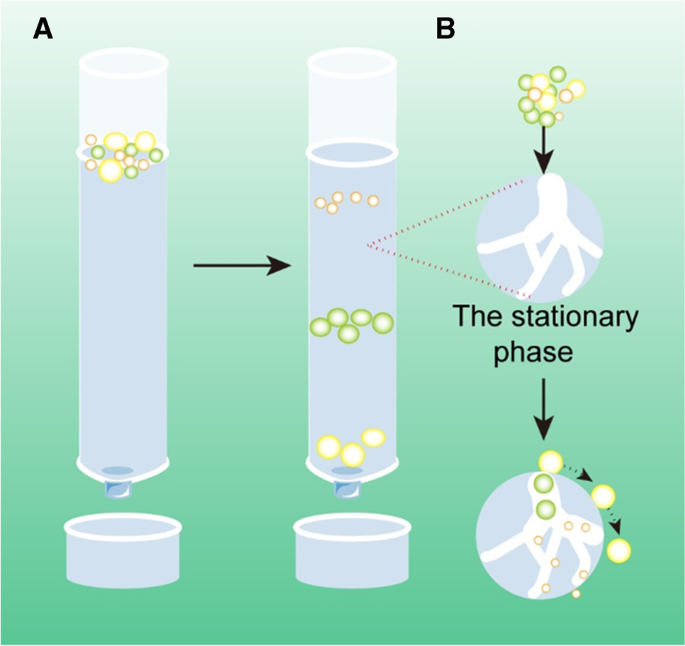The image is a detailed diagram with a green background that transitions from a lighter green at the top to a darker green at the bottom. At the top of the diagram, there are two labeled sections: A on the left and B on the right.

In section A, there is a vertical cylinder filled with blue liquid. Floating on top of this liquid are several spheres: four green, five red (referred to as orange in some descriptions), and three larger yellow ones. Beneath this cylinder is a bowl-shaped object. A black arrow points from this setup to the right, indicating a transition to section B.

Section B mirrors the structure of section A with another vertical cylinder containing blue liquid, but the spheres inside are now separated: five red spheres are at the top, five green spheres are in the middle, and three yellow spheres are at the bottom. This cylinder also has a bowl-shaped object beneath it.

To the right of section B, the diagram labels a process called "the stationary phase". This part of the diagram shows two large blue circles with white interiors. The top circle contains the red, green, and yellow spheres on its surface, while the bottom circle shows these colored spheres within the blue circle itself, more organized by size. Additionally, there are lines and arrows pointing out from these blue circles, indicating the sorting process.

The entire diagram illustrates a separation and sorting procedure, likely involving a stationary phase where various colored spheres are sorted by size as they transition from cylinder A to cylinder B and beyond.